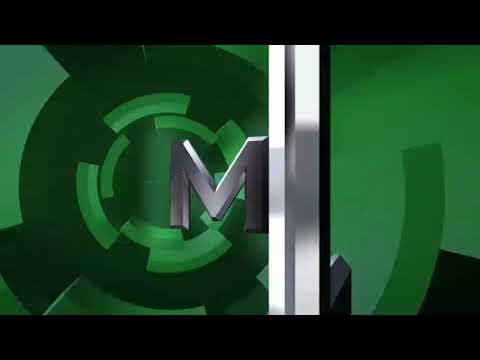The image features a predominantly green background with varying shades, including light, bright, and dark greens, giving a multi-dimensional appearance. On the left side, there is a circular design resembling a cogwheel, with an inner green circle bordered by a black outer circle. The foreground is dominated by a silver or grey metal rod, slightly right of center, extending vertically off the frame. Connected and jutting out to the left of this rod is a large, metallic, cartoonish capital letter "M". The entire setup suggests a stylized logo, potentially for a movie studio, set against a backdrop of detailed cogwheel shapes. The image is framed by black borders at the top and bottom, adding to its cinematic feel.